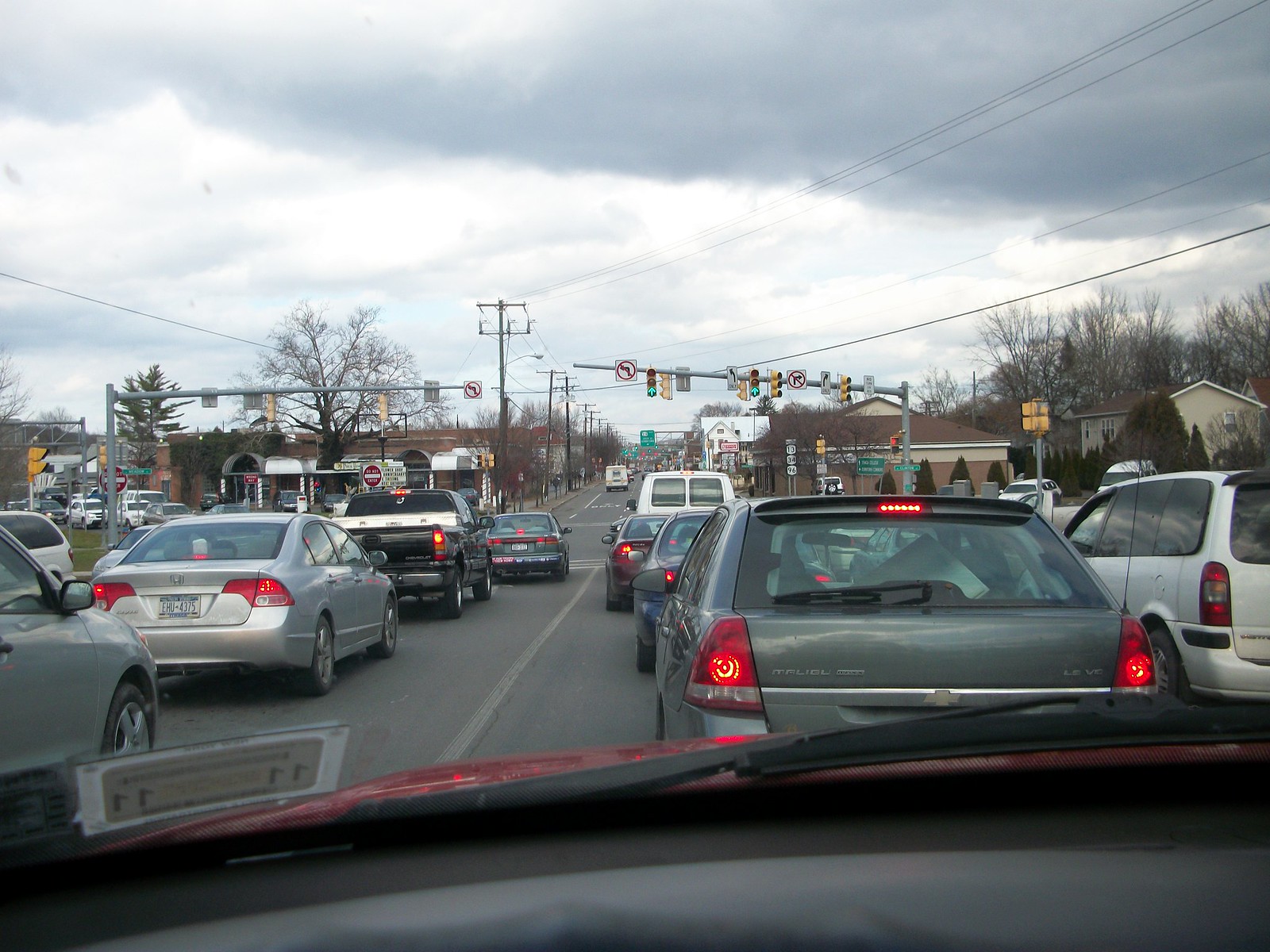The image captures a scene from inside a red vehicle, evidenced by the vehicle's red interior framing and black dashboard. A sticker is visible on the left-hand side of the window. The vehicle appears to be stuck in traffic, with the traffic light having just turned green. Street signs prominently display prohibitions for both left and right turns. Immediately ahead of the vehicle is a gray car, with another gray car to its left and a white car to its right. The sky above is overcast, suggesting impending rain.